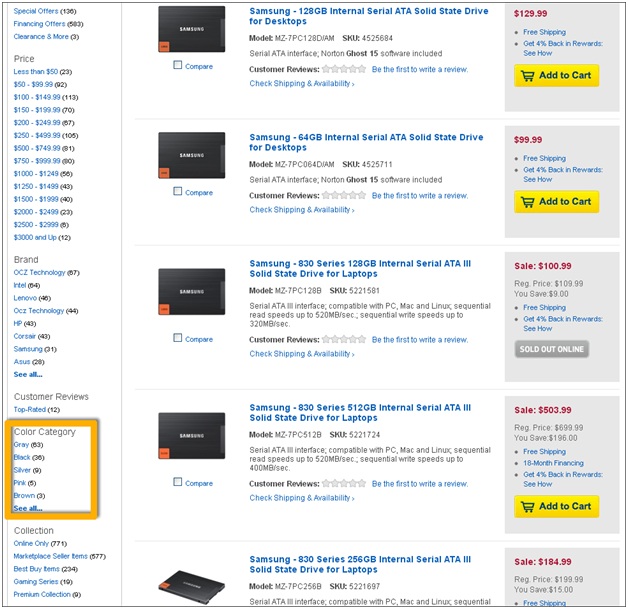The image illustrates a detailed comparison of Samsung Solid State Drives (SSDs) for laptops, taken from an e-commerce website. The central portion of the page lists five SSD options, each with distinct specifications and price points. Starting from the top:

1. A Samsung 12 GB SSD for desktops, priced at $129.99. It features a notation for free shipping and indicates a 4% rewards offer with a "See How" link. A prominent yellow rectangular button labeled "Add to Cart" is present.

2. Below it is a Samsung 16 GB SSD available for $99.99.

3. The third item is a Samsung 128 GB SSD from the 830 series, originally priced at $100.99 but currently marked as "Sold Out Online" in a gray box.

4. Next is a Samsung 830 series 512 GB SSD, which is listed for $503.99.

5. The final option is a Samsung 830 series 256 GB SSD, priced at $184.99.

Various other sections of the website are visible, indicating further browsing options or additional information.